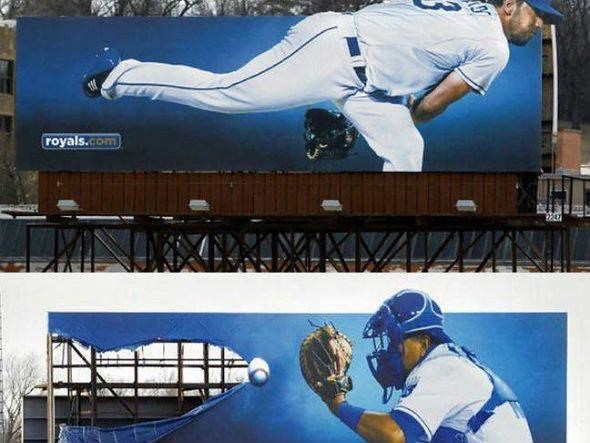These two vertically stacked images feature billboards. The top image showcases a billboard with a blue background and a brown lower section, displaying a baseball player dressed in white and blue. The player is in an action pose, leaning forward with his gloved arm positioned behind one of his legs. The text "Royals.com" is prominently displayed on this billboard.

The bottom image presents a damaged billboard with a significant portion missing, revealing the underlying wooden structure as well as the sky and some trees in the background. Despite the damage, the billboard's blue background remains visible. It depicts a baseball player preparing to catch a ball with a brown glove. The player wears a blue and white helmet, a blue and white shirt, and a noticeable blue object around his wrist and another device on his back. The quality of the bottom image is somewhat grainy, adding a layer of visual texture to the scene.